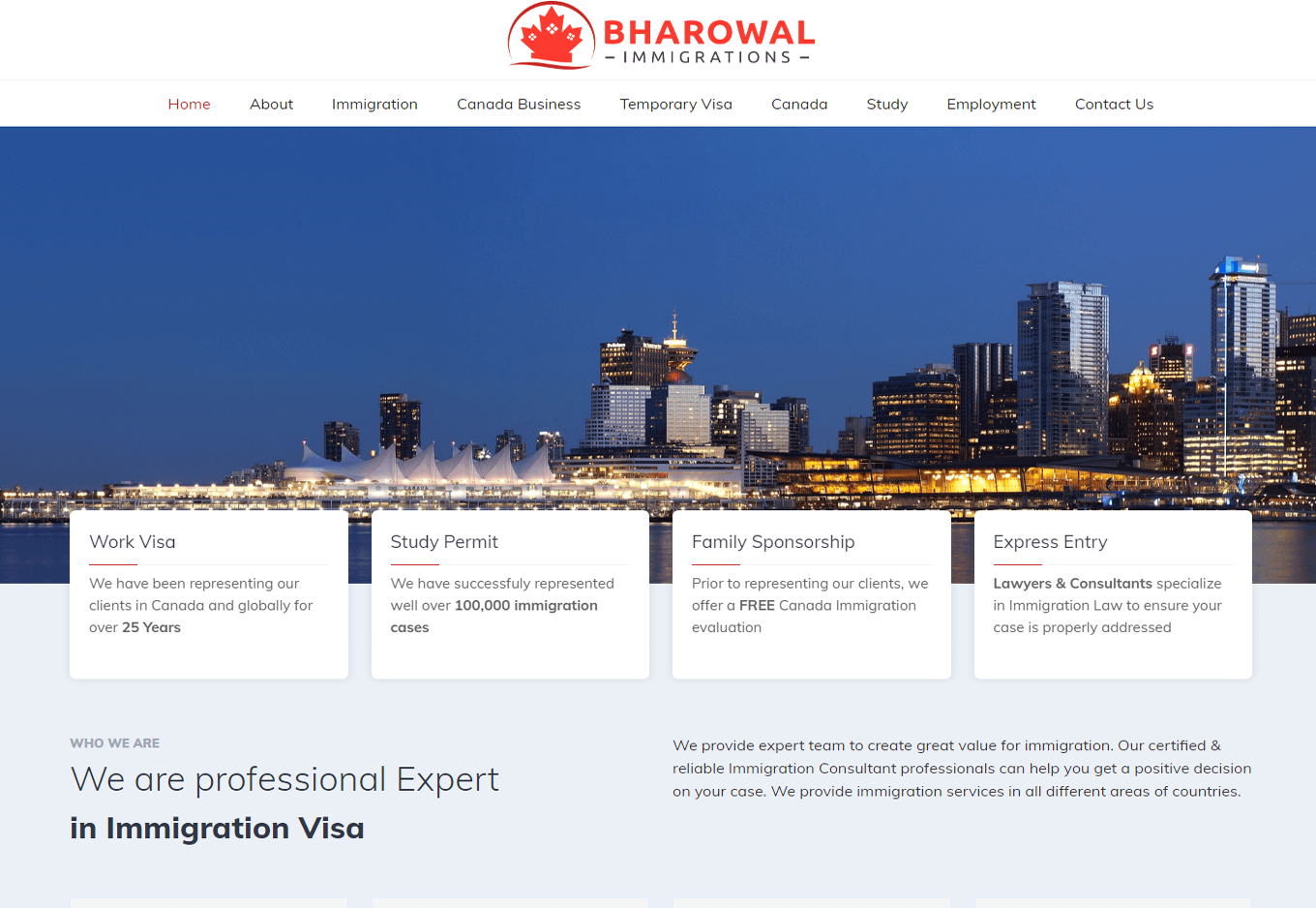The website for "Bravo Immigrations" prominently features a sleek design that begins with a striking red logo, adorned with a leaf, followed by the firm’s name. The navigation bar is conveniently located beneath the logo and offers the following options: Home, About Immigration, Canada Business, Temporary Visa, Canada, Study, Employment, and Contact Us.

Centrally displayed is a large, captivating image of what appears to be the Toronto cityscape, establishing the Canadian focus of the site. Below this image, the website provides detailed information about its services. The sections include "Work Visa" which boasts 25 years of global representation experience, "Study Permit" that highlights their success in over 100,000 immigration cases, and "Family Sponsorship", emphasizing a free Canada immigration evaluation service. Another section, "Express Entry," mentions that they have specialized lawyers and consultants dedicated to effectively addressing immigration cases.

Towards the bottom, the site introduces the firm and its ethos under "Who We Are". The text explains that Bravo Immigrations prides itself on its professional and expert team, aimed at delivering immense value in the realm of immigration. It reassures potential clients of their certified and reliable immigration counsel professionals, committed to securing positive decisions. The firm offers comprehensive immigration services across various countries, emphasizing their global reach and expertise.